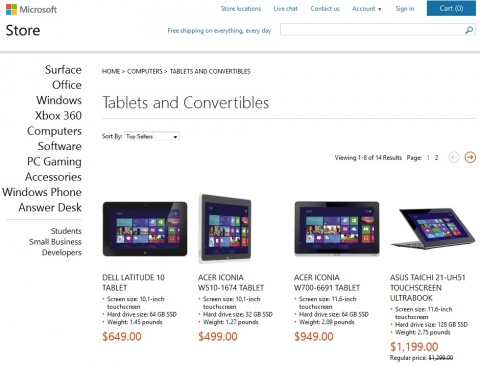This image is a detailed screenshot of the Microsoft online store interface. At the top left corner, the recognizable Microsoft logo with squares in red, blue, green, and yellow is prominently displayed next to the "Microsoft" text. Across the top horizontal menu bar, written in blue letters, are several navigation tabs including "Store," "Location," "Live Chat," "Contact Us," "Account" (which is a dropdown menu), "Sign In," and a blue "Cart" button with white letters indicating zero items in the cart.

Just below, in bold black letters, the word "Store" is prominently displayed. Adjacent to it, a blue text line states "Free shipping on everything, every day." A white search bar with a blue search icon is placed beneath this line, separated by a gray line from the rest of the page.

On the left sidebar, a list of clickable categories is presented: "Surface," "Office," "Windows," "Xbox 360," "Computers," "Software," "PC Gaming," "Accessories," "Windows Phone," and "Answer Desk." Below a gray divider, additional categories listed are "Students," "Small Business," and "Developers."

In the central section, bold black letters announce "Tablets and Convertibles," showcasing four tablet options: two from Dell, two from Acer, and one from Asus.